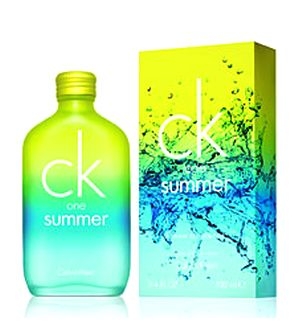The image features a bottle of Calvin Klein cologne alongside its packaging. The bottle is constructed of glass and showcases a vibrant, multi-colored design. It has a twist-off metal lid that is neon yellow. The glass body transitions from a neon yellow at the top, to neon green, then a darker turquoise, and finally a lighter turquoise at the bottom. Prominently displayed at the top of the bottle is a large, white CK logo for Calvin Klein. Below this, in smaller white letters, is the word "one", followed by the word "summer" in a slightly larger white font.

The accompanying box is rectangular and made of cardboard, designed to house the bottle securely. The top of the box features a neon yellow hue, flowing down into shades of neon green, turquoise, blue, and lighter turquoise. The box is artistically adorned with lines depicting water splashes in varying hues of blue and darker green. The CK logo in off-white is positioned at the top of the box, with "one" in small white letters underneath and "summer" in a slightly larger white font. This energetic and colorful design captures the essence of the Calvin Klein One Summer fragrance.